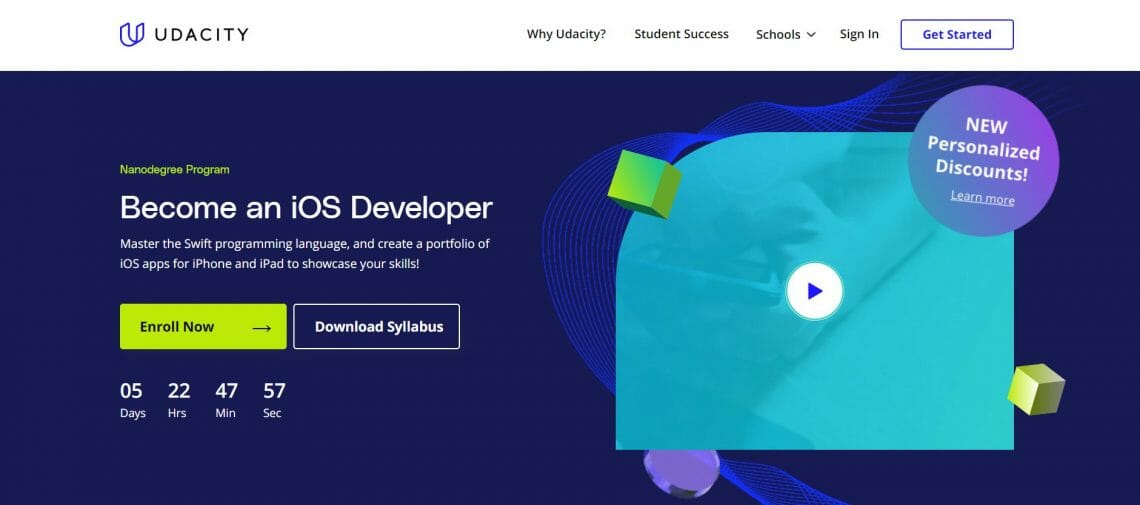The image is a screenshot from the website "Udacity" (U-D-A-C-I-T-Y). At the top left corner, there is a three-dimensional, stylized letter "U" serving as the site's logo. The header includes navigation options: "Why Udacity," "Student Success," "Schools," "Sign In," and "Get Started."

Dominating the middle section of the screenshot, the background shifts to a deep navy blue. Over this backdrop, in vibrant neon green text, the following information is displayed: "Nano Degree Program: Become an iOS Developer, Master the Swift Programming Language, and Create a Portfolio of iOS Apps for iPhone and iPad to Showcase Your Skills." Below this description, there is a conspicuous neon green button bearing the text "Enroll Now." An arrow directs the viewer's attention towards a link that reads "Download Syllabus."

Towards the bottom of the image, a countdown timer in white text indicates a remaining duration of five days, 22 hours, 47 minutes, and 57 seconds. This is likely the time left to enroll or access a particular offer related to the Nano Degree program.